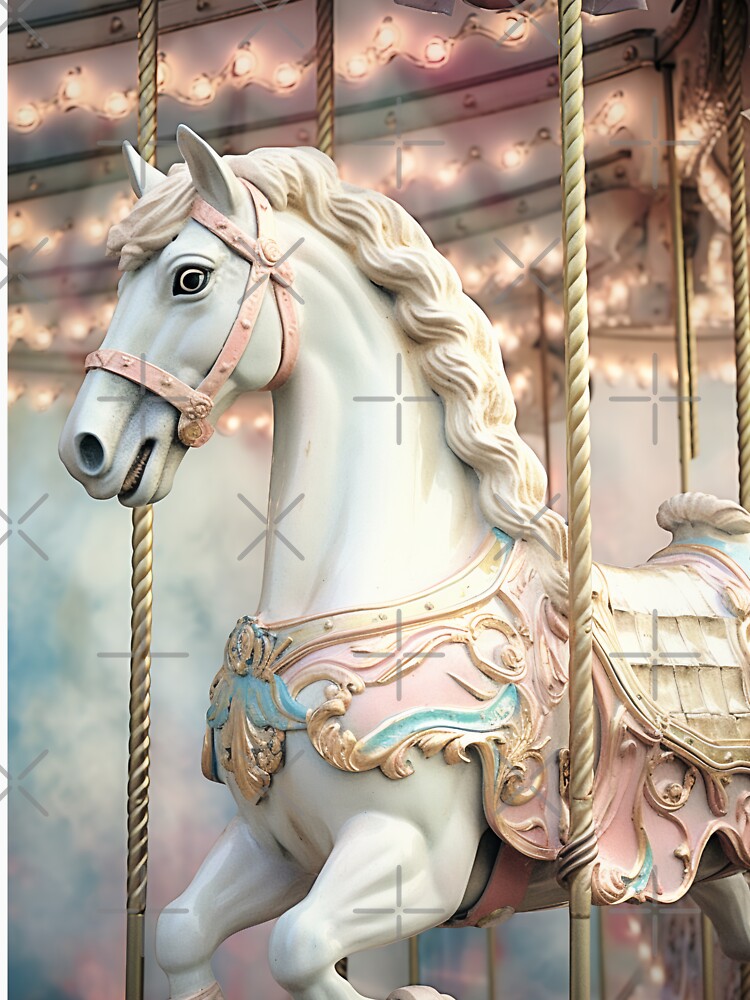In broad daylight, this image captures a dazzling carousel horse at an amusement fair, overlaid with a watermark comprised of intersecting gray lines forming X's and a plus sign, accompanied by scattered dashes. The scene reveals a meticulously detailed, shiny white horse crafted from either fiberglass or plastic. Adorned with an elegant pink bridle around its face and a decorative pink breastplate embedded with intricate flower engravings, the horse sits proudly on a spiral-patterned gold pole that extends from top to bottom. The horse, facing left, features carefully painted black eyes with white accents, a mouth ajar revealing white teeth, and a luxurious white mane. Behind the horse, the carousel’s gleaming lights and vibrant colors such as turquoise, pink, and gold create a lively background, with numerous yellowish lights illuminating the top. This mesmerizing figure, complete with a gold-colored saddle showcasing a patchwork-like seat, epitomizes the enchanting charm of a traditional fairground ride.